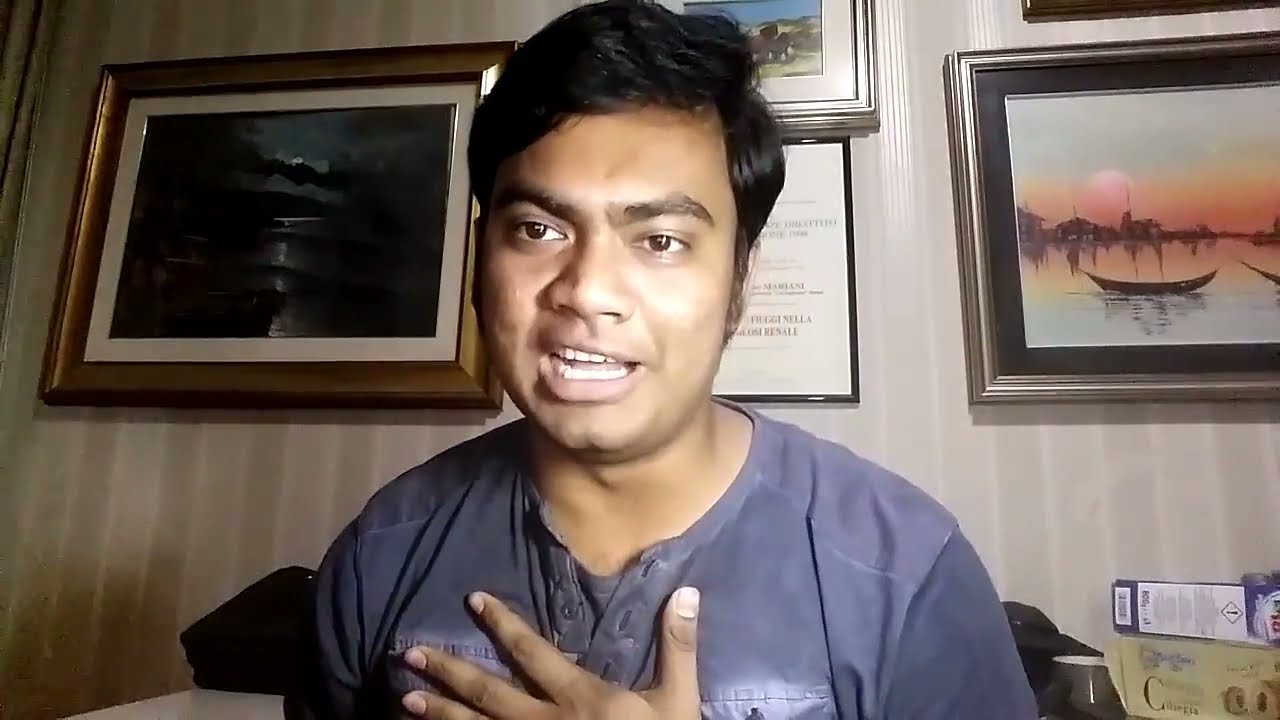In this image, we observe a man of potential Middle Eastern or Indian descent positioned centrally and gazing directly at the camera, as if in mid-conversation, with his right hand placed on his chest. He has black, slightly parted hair and well-defined black eyebrows, and is dressed in a blue shirt with a buttoned collar, which appears darker on the sleeves. The setting seems to be indoors, possibly in his office or home, featuring tan and white-colored walls. Behind him are several framed artworks: to the right, a painting of wooden boats resting in water against a sunset backdrop, casting an orange and yellow hue; to the left, another painting depicting boats under a dark, cloudy night sky illuminated by a glimmer of moonlight. Additionally, directly above his head, there is a framed document that looks like a diploma or certificate. The lower right corner of the image shows some packages, and there is also a cup on a table. The overall image conveys a cozy, personal space with a touch of professional ambiance.